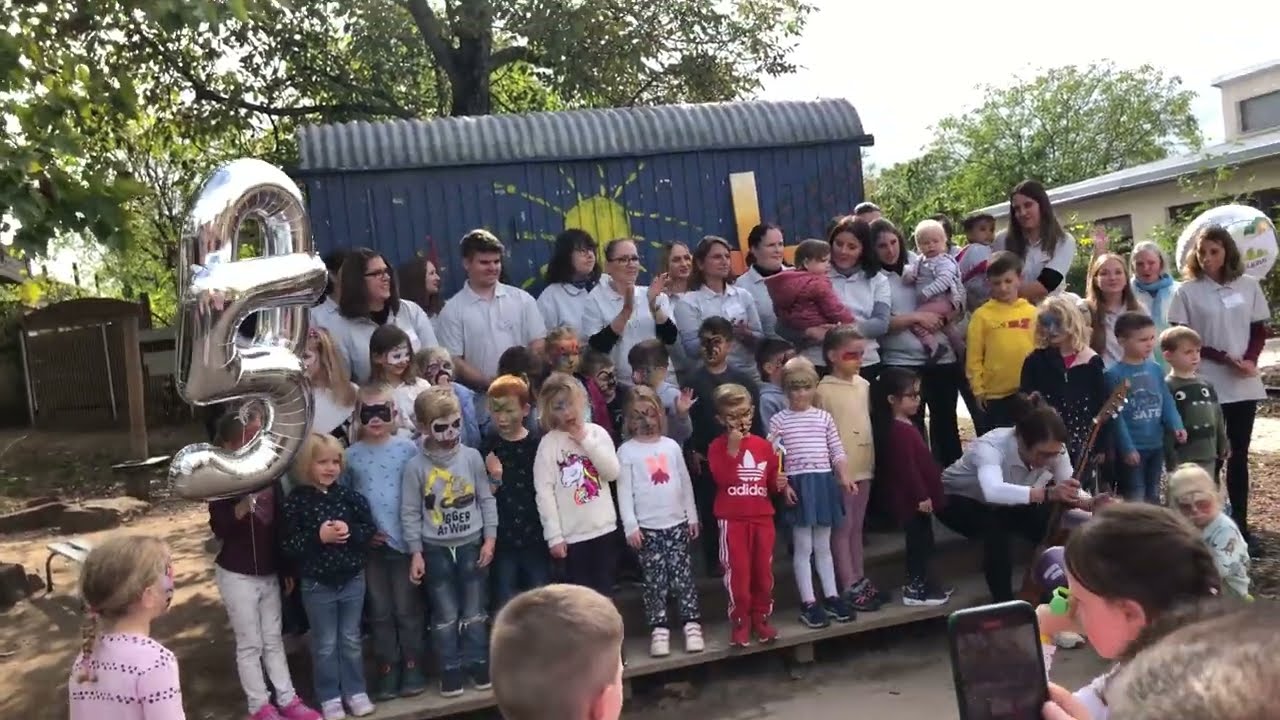The image captures a lively outdoor scene where a large group of children and adults are gathered, posing on a set of outdoor stairs or bleachers in front of a blue, metal structure adorned with a painted yellow sun. In the front rows, about 20-30 children, appearing around five to six years old, are dressed in uniforms or polo shirts. Behind them stand adults, some cradling babies, creating a familial, festive atmosphere. Large metallic balloons displaying the number "50" suggest a celebratory occasion, likely a 50th anniversary or birthday. The scene is brightly lit by daylight filtering through the surrounding green trees, under a partially overcast sky. There are additional structures in the background, including a cream-colored building with a gray roof and a tin shed with a light blue roof, blending harmoniously with the natural setting. Onlookers are seen to the right, some capturing the moment with their cell phones, adding to the vivacious spirit of the gathering.